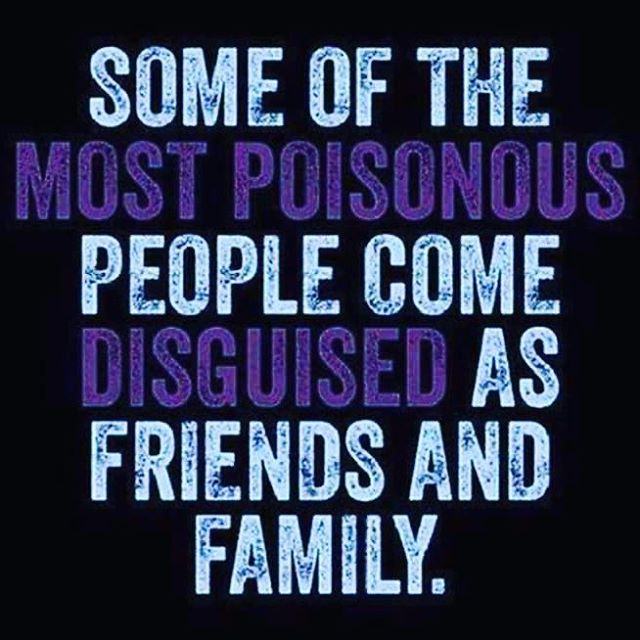The image features a quote presented on a dark blue, almost black background. The text of the quote reads, "Some of the most poisonous people come disguised as friends and family," and is entirely capitalized in a condensed sans serif font. Most of the words are in light blue, adorned with a subtle splotchy texture for added visual interest. The words "the most poisonous" and "disguised" stand out prominently in dark blue or dark purple, emphasizing their significance within the quote. This visually striking design is commonly used for social media sharing, aiming to convey its poignant message effectively.